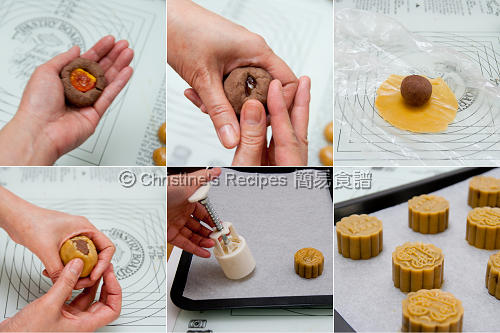This detailed six-image collage from "Christine's Recipes" showcases the step-by-step process of making traditional mooncakes. The collage is arranged in a vertical rectangle with three images on the top row and three on the bottom. The background features a white paper with black circle patterns.

1. **Top Left Image:** A hand holds a thick, round piece of dark brown dough with a red filling in the center.
2. **Top Middle Image:** The dough is pinched closed around the red filling, transforming it into a ball.
3. **Top Right Image:** The ball of dough is placed on a small yellow pancake-like pastry.
4. **Bottom Left Image:** The yellow pastry is then wrapped around the brown dough ball, shown being held by two hands.
5. **Bottom Middle Image:** A white device, possibly a mooncake mold, presses down on the wrapped ball, forming intricate designs on the pastry.
6. **Bottom Right Image:** The final image displays several neatly designed mooncakes on a cookie sheet, ready to be baked.

Above the collage, a watermark reads "Christine's Recipes" alongside four Chinese characters, indicating the cultural origin of the recipe.